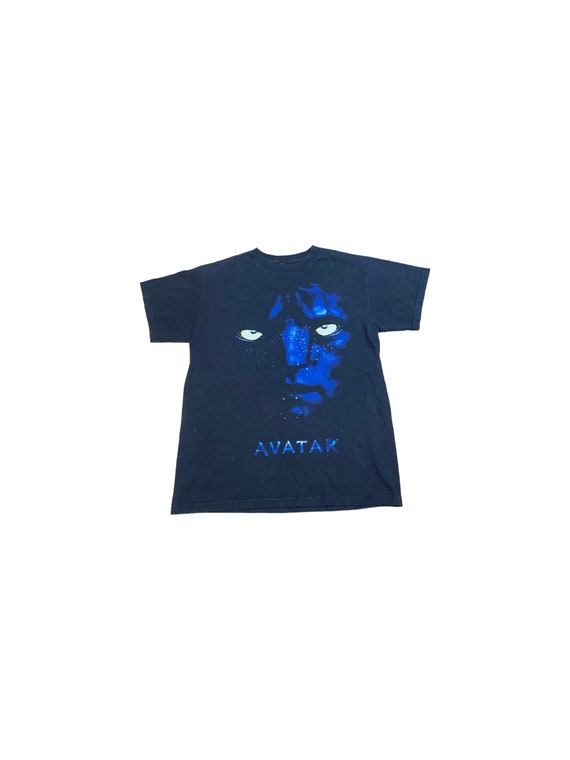The image presents a detailed photograph of a navy-colored t-shirt, laid flat with its arms outstretched, occupying the entirety of a white background. The t-shirt showcases a prominent design related to the movie "Avatar." Centered on the shirt is the half-lit, half-shadowed face of a Na'vi character with distinct blue skin and piercing yellow eyes, staring intensely ahead. Notably, the left side of the face is more visible, while only the eye is discernible on the right side. Below the face, the word "Avatar" is emblazoned in striking blue lettering. The shirt appears to be sized for a child, though the exact dimensions are difficult to ascertain from the photo. The image focuses solely on the shirt without any additional elements or text.